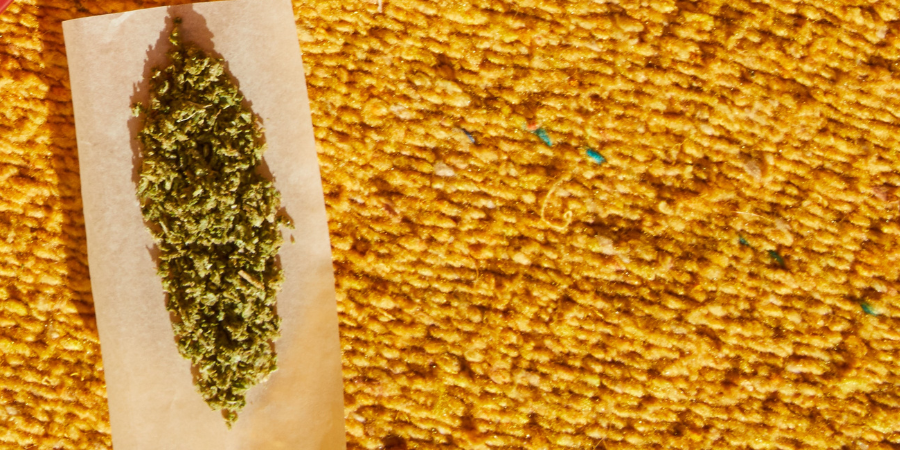The image captures a close-up shot taken from above, showcasing a mustard-colored shag carpet that forms the background. On the left side of the carpet, a rectangular sheet of white rolling paper is laid out neatly. Positioned at the center of this paper is a mound of dried, green-and-brown marijuana, orderly placed and ready for rolling. The texture and color details, including the vibrant mustard carpet and the white paper contrasted with the greenish-brown marijuana, create an intricate and detailed composition. It appears that someone is preparing to roll the marijuana into a joint, possibly pausing to admire or document their setup.